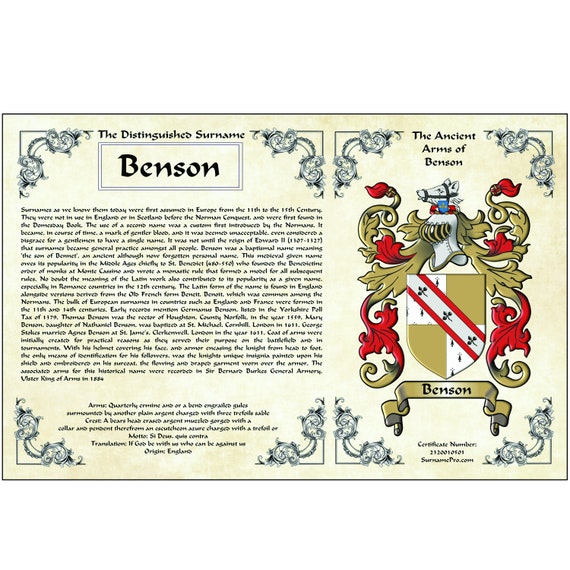This landscape-oriented image features a detailed illustration accompanied by text on the left-hand side. Enclosed within a rectangle adorned with ornate scrollwork at each corner, the prominent black text reads "The Distinguished Surname Benson." Below this headline lies a passage of smaller, mostly unreadable text, beginning with "Surnames as we know them were first assumed in Europe from the 10th to the 15th century."

On the right-hand side, the image showcases an intricate coat of arms. At the top, a helmet supports an animal's head, which could be a horse or dog. The background behind the helmet features swirling, decorative designs. Below, a shield is divided into four quadrants: the lower left and upper right are tan, while the upper left and lower right are white with a recurring pattern. A diagonal white band, edged in red and decorated with a black pattern, spans from the upper left to the lower right quadrant. Completing the coat of arms is a scroll beneath the shield, inscribed with the name "Benson." The image, rich in colors including tan, white, red, black, and a hint of blue, appears to be part of a heritage certificate or pamphlet, likely detailing the historical significance and lineage of the Benson surname.